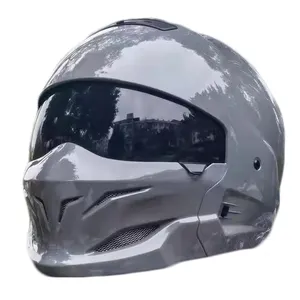The image depicts a highly detailed, up-close view of a motorcycle helmet, centrally placed within a square frame. The helmet is diagonally oriented, facing toward the left-hand corner of the viewer. It features a gleaming silver exterior that vividly reflects its surroundings, including trees and buildings. The top of the helmet is rounded, featuring a prominent black strip or latch. Below this, the visor area is dark and opaque, effectively mirroring the nearby elements. The mouth section showcases multiple grill openings to facilitate breathing. Additionally, there are small black spots, possibly bolts, noticeable on the right side of the helmet. The sleek, modern design of the helmet stands out against a stark white background, making it appear as either a high-definition photograph or a modern art illustration.